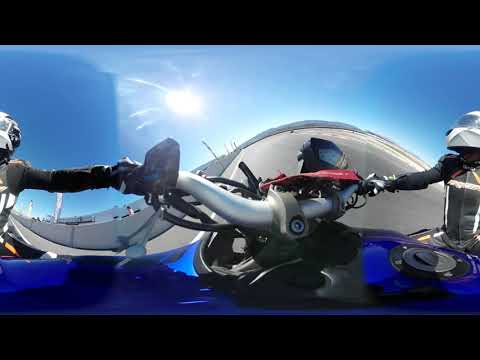The image captures a dramatic fisheye lens view of a motorbike racing scene under a radiant blue sky with the yellow sun shining brightly. The central focus is on a blue motorbike with a black gas cap, its chrome and metal handlebars distorting into the curvature of the lens. A rider, clad in a leather motorbike suit adorned with gray, white, and yellow stripes, grips the handlebars. Their gray helmet and the specialized racing suit suggest a professional setting, likely a race track conveyed by the track border seen in the distance. The fisheye effect creates a surreal image where the rider appears split, magnifying the handlebars at the center and warping their arms and suit. The clear outdoor setting highlights the stark contrast between the vivid blue sky and the metallic and leather textures of the motorbike and the rider.